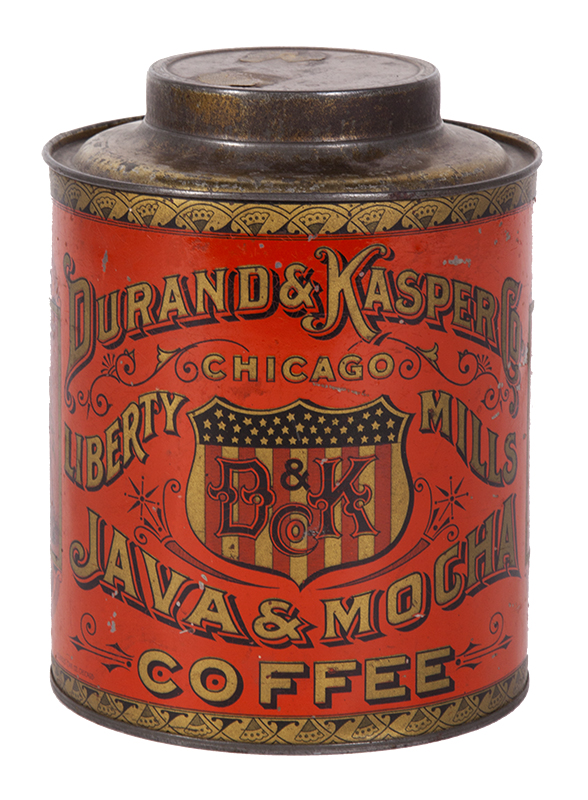This close-up image showcases an antique, weathered coffee can made of bronze-colored metal. The can, likely from the 1800s, has a distinctive red background with gold and black trim. It bears a highly detailed, ornate label with gold serif lettering that reads: "Durand and Casper, Chicago, Liberty Mills, Java and Mocha Coffee". The centerpiece of the can is a logo featuring a crest reminiscent of the American flag, with red and white vertical stripes and a dark blackish-blue top adorned with white stars, containing the initials "D and K". The lid of the can appears to be metal, with a mix of dark black and a faded goldish tint, designed to twist on and off. The overall condition of the can is quite worn, enhancing its antique charm. The can is set against a plain white backdrop, which highlights its aged beauty and intricate design.